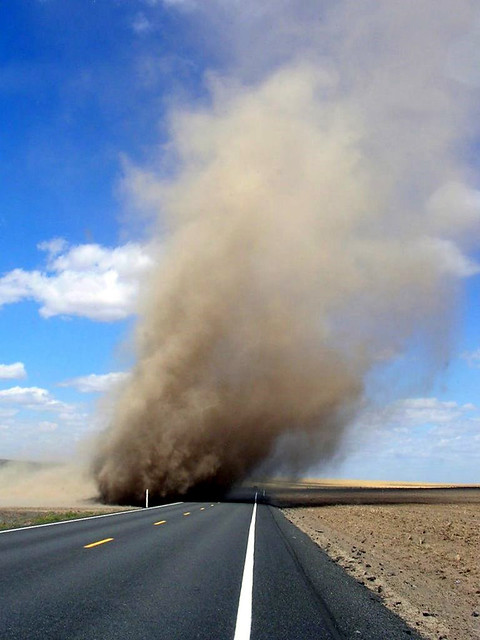The photograph captures a straight, newly paved black tarmac road with two lanes separated by a dashed yellow divider, and solid white lines marking the outer boundaries. The road stretches into an arid desert landscape characterized by barren, brownish rock and dust, with flat, tree-less terrain on either side. Dominating the scene is a large dust devil, a swirling wind pattern stirring up clouds of brownish-yellow dust. This dust devil, appearing massive and significant, is either just crossing or about to cross the road, overlapping slightly with it yet leaving the surface clear. The bright blue sky with scattered white clouds forms a vivid backdrop, and the dust devil casts a discernible dark shadow on the dry ground, accentuating its presence. The right side of the image reveals more dirt and open fields, highlighting the expansive, desolate environment.